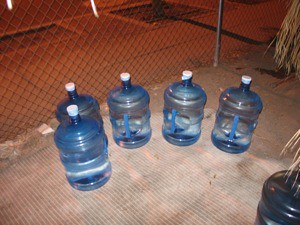This is a photograph taken outdoors at night, depicting five large blue plastic water jugs with white caps and handles, typically used in water dispensers seen in offices. The jugs are situated near a silver chain-link fence, beyond which there is a sidewalk with sections of dirt for planters, all cast in a red-orange streetlight. The ground is concrete, appearing grayish under the white lighting but turning reddish outdoors due to the streetlight. A striped rug lies beneath the jugs, indicating they are resting on this rather than directly on the concrete. In the lower right corner of the image, there is a dark, seemingly empty jug. To the right, there are yellow, dead-looking palm fronds or grasses. The photograph captures an alleyway scene with the jugs clearly visible against the backdrop of the fence and illuminated pavement.